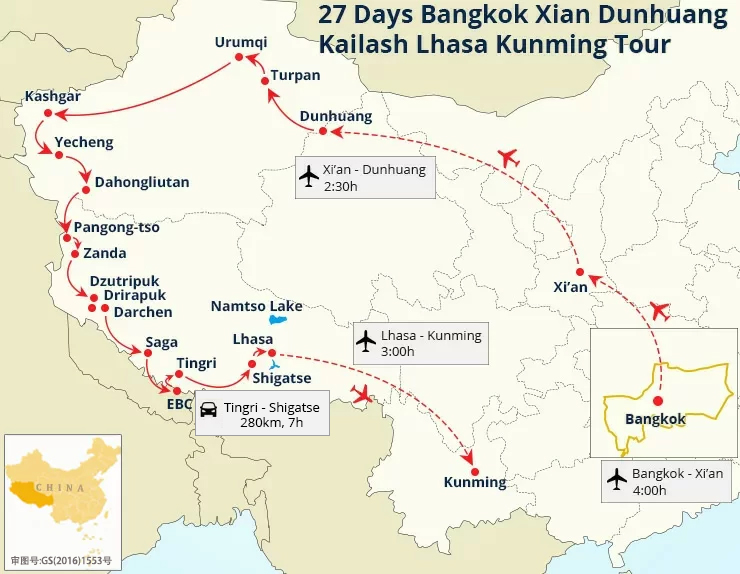The image depicts a detailed travel map showcasing a 27-day tour from Bangkok to various cities in China. At the top, the caption reads "27 days Bangkok, Xi'an, Dunhuang, Kailash, Lhasa, Kunming tour." The primary map is beige and tan, featuring blue edging at the bottom to represent water. A series of red solid and dashed lines trace the flight path, starting from Bangkok and moving across multiple cities in China, such as Xi'an, Dunhuang, Turpan, Urumqi, Kashgar, Lhasa, and finally Kunming, with red airplane icons marking each flight segment. 

In the bottom left corner, an inset displays a yellow outline of China labeled "China," with the southwestern region colored darker, emphasizing the tour's route. Another inset in the bottom right corner features a black square with a yellow country outline and a red dot marking Bangkok, indicating the flight's origin from Thailand to China. The map itself uses a white color to depict China, with bordering countries shaded in tan, providing a clear distinction between the regions. Detailed black text labels the cities along the tour route, enhancing the overall readability and comprehensiveness of the travel itinerary.